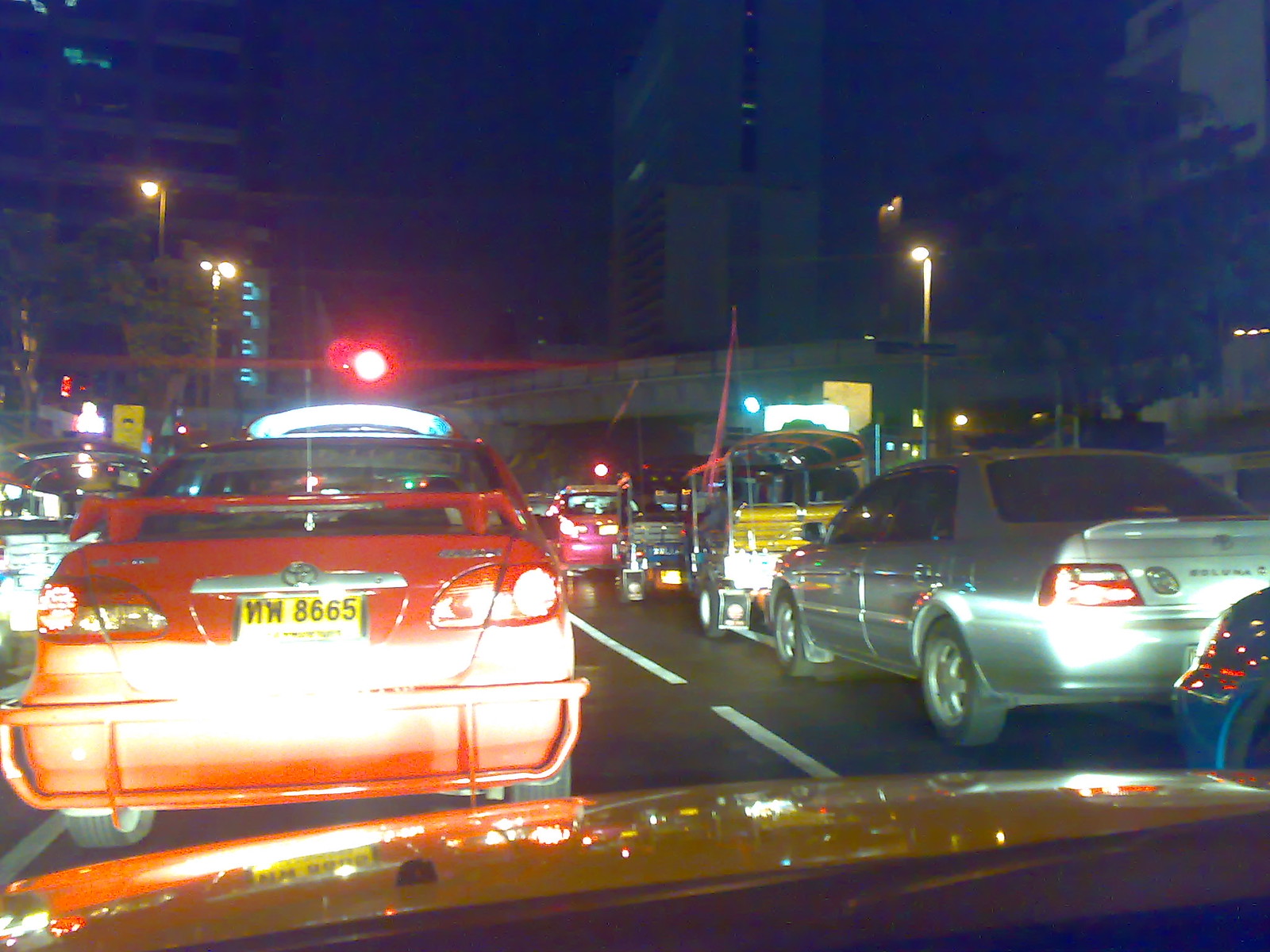A bustling urban night scene captured from inside a vehicle, possibly a yellow taxi, at a red light in the heart of a city. The street is enveloped by towering skyscrapers, their tops obscured from view, likely serving as both apartment and office buildings. The vehicle is surrounded by an assortment of cars, including a red sports car directly ahead, distinguished by its rear spoiler and a license plate reading NW8665. To the left, a partial view reveals a sequence of vehicles: a blue car, a silver one, a truck or jitney, and another red car further up. Streetlamps illuminate the scene, highlighting the congested yet static nature of the moment at the red light.